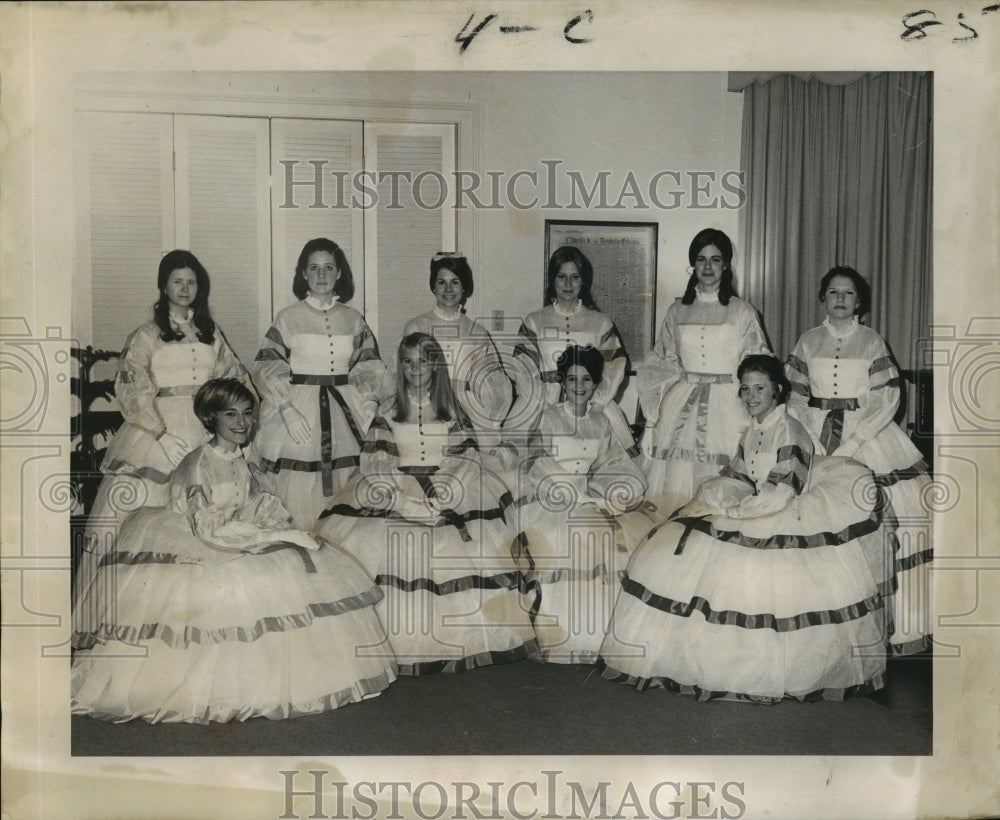This historical black-and-white photo, prominently watermarked with "Historic Images" twice—once near the top and once near the bottom—depicts a formal gathering of ten young white women, likely from the early 20th century, possibly the 1920s. The image, bearing the code "4C85" on its white border, features women dressed in elaborate, identical gowns. These dresses are characterized by large hoop skirts adorned with multiple horizontal ribbons at the hem and layers, high collars, and numerous buttons running down from the neckline to a ribboned waist. The top part of the dresses has sheer sections between the collars and the bustlines, with the rest being solid fabric. The sleeves are similarly poofy with ribbons and are sheer from the high collar to the bustline. Four of the women are seated, while the remaining six stand behind them, all posing in front of a backdrop of grayish curtains with a barely discernible photo and a closed closet in view—elements contributing to an antique atmosphere. The central figure, distinctively dressed without ribbons, suggests a special role, possibly indicating a debutante gathering or a wedding party.